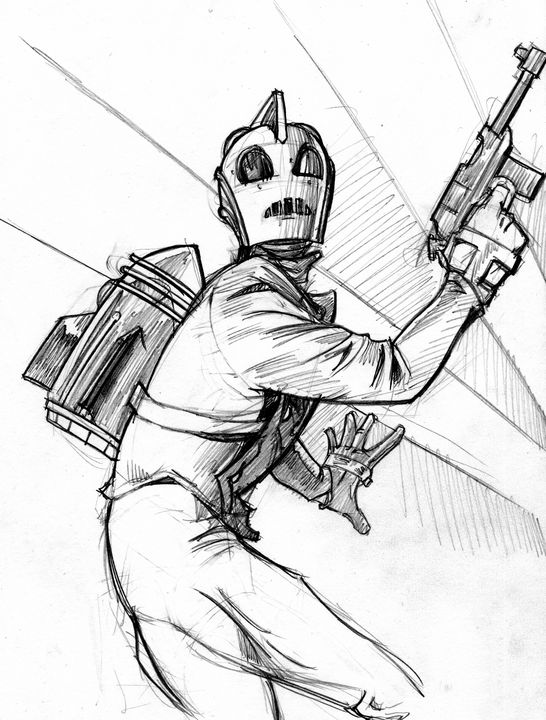The sketched image depicts a figure dressed in a white jumpsuit and wearing a silver, robot-like helmet that completely covers their face. The character, slightly bent forward, is holding a machine gun in their right hand, which is raised and aimed towards the upper right part of the image. Their left hand is outstretched in front of them, palm outward as if pressing up against something or bracing. A backpack resembling a jetpack with a triangular, rocket-like tip is strapped to their back, complete with visible straps extending from the chest to the back. The sketched background features alternating diagonal lines and squiggly filled-in sections on a white backdrop, giving an impression of movement or action emanating from the right side. The person in the sketch appears to be staring straight ahead with a tense and possibly startled expression, suggested by the filled-in dark shapes of the eyes and mouth on the helmet. The overall aesthetic is a detailed pencil drawing with a brownish-black or gray tinge against a white background, suggesting a dynamic and possibly futuristic or space-themed scenario.